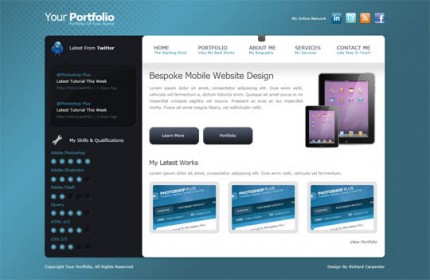The background of the square is a soothing teal blue. In the top left corner, the text "Your Portfolio" is prominently displayed. Below this heading, a long black rectangle features a small blue circle at the top, containing tiny white text. Adjacent to the blue circle, there's a white wrench icon, next to which the text "My Skills and Qualifications" is written in white. Additionally, several rows of blue stars decorate the area beneath.

On the right side, enclosed within a white box, are navigation options listed at the top: Home, Portfolio, About Me, Services, and Contact Me. Directly below this section, text reads "Bespoke Mobile Website Design" and showcases two black iPads. The screens of these iPads have a purple hue and display multiple app icons arranged in rows. To the left of this, there is a black box with the option to click "Learn More."

At the bottom of the design, the phrase "My Latest Works" is written in black text. Beneath this, three clickable squares are shown, each with a blue background and small areas of white text.